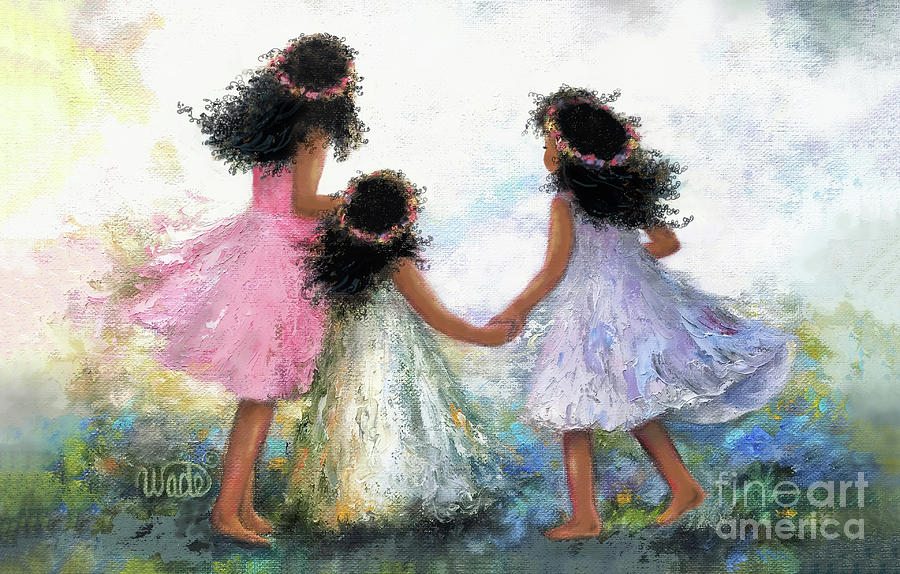This painting, likely a mix of watercolor and acrylic, depicts three young Black girls, possibly sisters, standing hand-in-hand in a grassy field under a bright daytime sky. Their backs are to the viewer, revealing only their dark, long, curly hair adorned with crowns of flowers. The leftmost girl, the tallest, wears a flowing pink dress. The middle girl, the shortest, is dressed in a floor-length light green gown. The rightmost girl, about as tall as the girl on the left, wears an elegant purple dress with blue and lavender hues. The background is a soft, sponge-painted blend of grayish-white with hints of yellow, suggesting they are gazing into the horizon. The painting carries the text "Wade" and "Fine Art America," indicating the artist and platform. The girls are barefoot, and the piece exquisitely captures their innocence and the beauty of their connection.